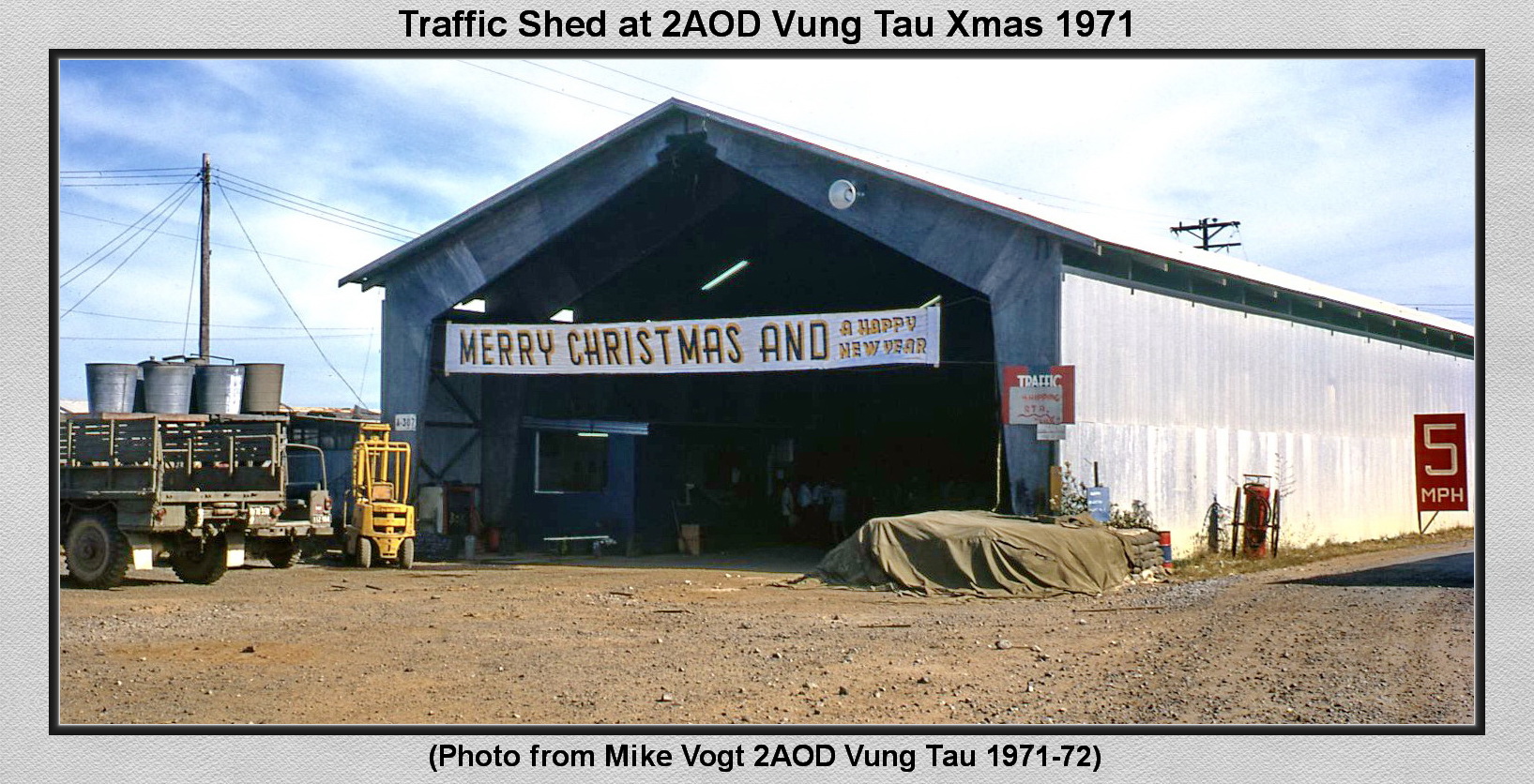The image is a color photograph taken during the Vietnam War, specifically at the "Traffic Shed at 2AOD Vung Thao, Xmas, 1971," with the photo credited to Mike Boyd. The large, silver metal shed prominently displays a banner that reads "Merry Christmas and a Happy New Year," signaling a festive attempt by the soldiers during the holiday season. The shed is situated in a barren, desert-like environment with no grass, only brown dirt. Several pieces of military equipment are visible, including trucks and a loader machine stacked with supplies, possibly oil gallons, which are parked nearby. There are also power lines in the background, and a gray or brown tarp covering something next to the building. Additionally, a "5 miles per hour" speed limit sign is visible on the right. The shed appears to be part of a larger logistical operation, serving as a storage or supply depot, and it's implied that soldiers might be inside, possibly preparing for a holiday gathering. Notably, the photograph captures a bright, sunny day with some clouds in the sky.